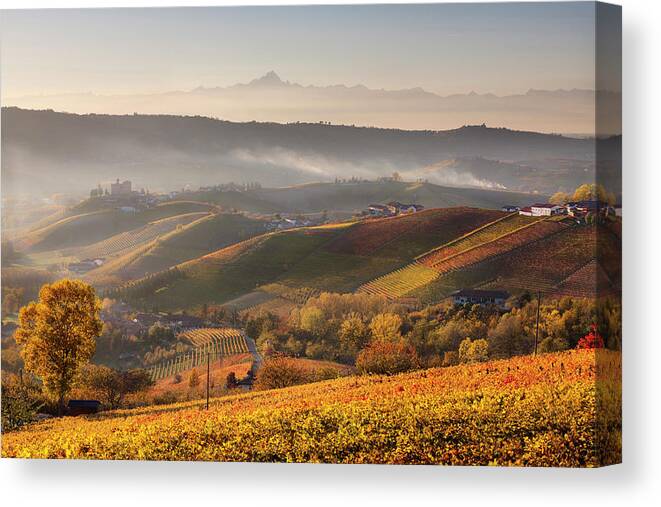In this detailed and vibrant painting, a rectangular canvas showcases an overhead view of a rolling, autumnal landscape. The grainy, low-definition image beautifully captures sprawling plains with golden grasses and colorful shrubs cascading over the hills. Amidst this picturesque setting, there are distinct patches of farmland, autumn harvest hues of red, brown, and yellow, and a scattering of green trees and bushes.

The sun sets from the left, casting a warm, golden light over the scene, enhancing the fall colors and giving the entire panorama a serene, glowing effect. Nestled atop the hills are quaint houses and buildings, suggesting a peaceful farming community. In the distance, majestic mountains rise, lightly veiled by fog, with a blue, foggy sky that adds depth and texture to the background.

The painting's three-dimensional look is accentuated by shadowing on the right side, giving the impression of depth and realism. It beautifully marries nature's raw beauty with a touch of human presence, celebrating the spectacular colors and tranquil ambiance of the fall season.